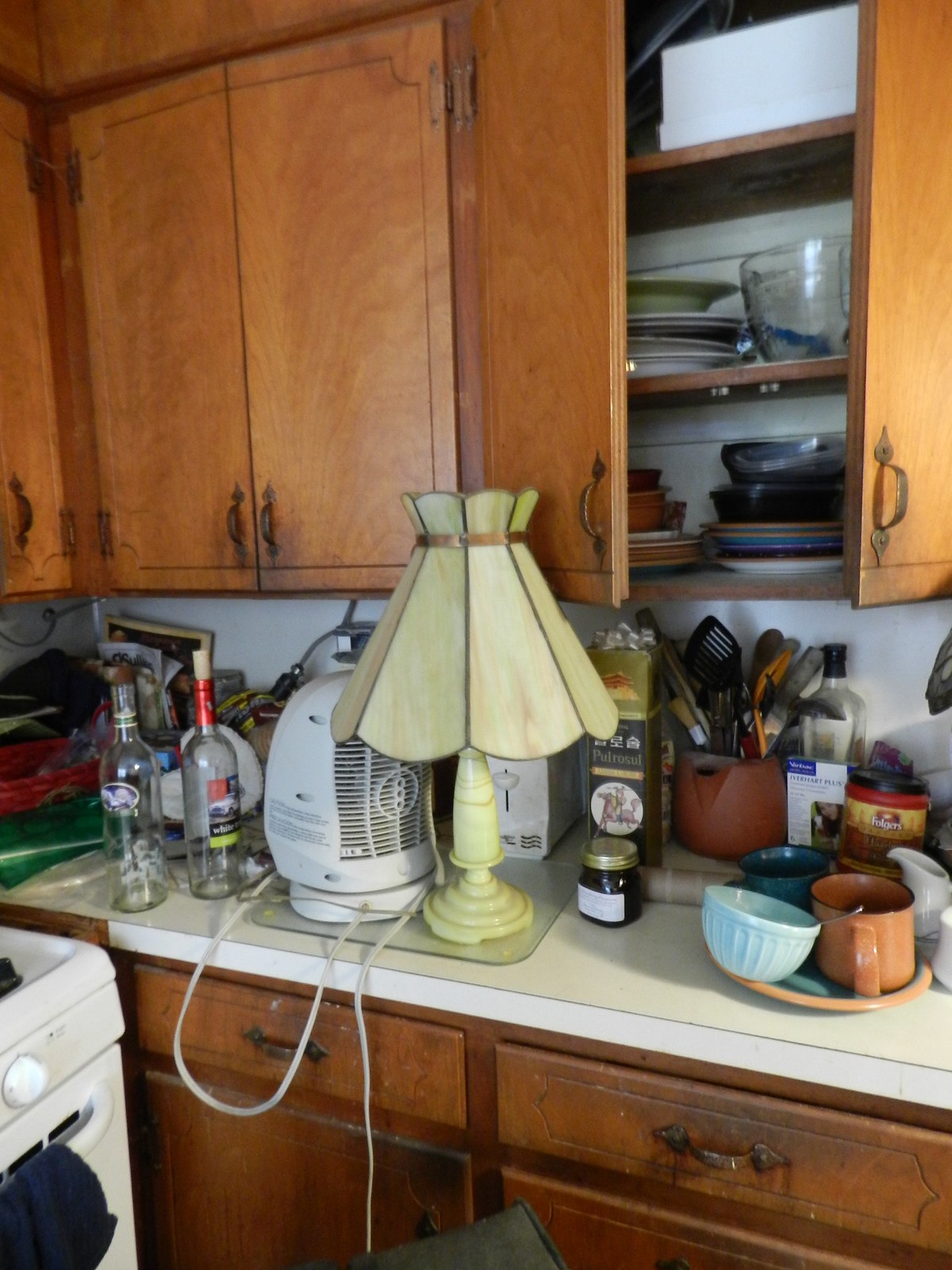In the image, we observe a cozy yet cluttered kitchen scene. The countertop is crowded with various items, indicative of an active cooking space. To the left, there is a white stove with a towel hanging on the handle and a small section of the front burner visible. Adjacent to the stove, several items are arranged on the countertop, leading towards the corner.

Among these items are two empty bottles that once contained alcoholic beverages. A small fan and an old-fashioned beige lamp are positioned nearby. There's also a jar, possibly containing some type of marinade. Behind the lamp, another small appliance is partially obscured by the lamp's shade.

An arrangement of cooking utensils, including a spatula and a ladle, is housed in a container on the counter. Additionally, a plate is set with a bowl resting on it and two mugs. On the far right of the countertop sits a coffee canister.

Below the cluttered countertop are several drawers with brown handles, and cabinets line the space above. Two of these cabinets are closed while one is open, revealing a stack of dishes, predominantly plates, a couple of bowls, and a large measuring cup. There is also an additional unidentified bottle situated slightly behind the coffee canister.